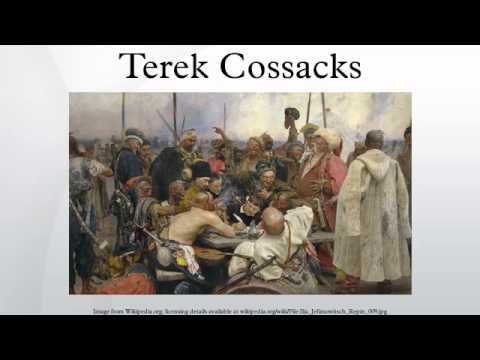The image features a historical scene depicted in a rectangular oil painting titled "Terek Cossacks," with the title in black letters at the top. The painting is framed with a white border and flanked by black stripes at the top and bottom. Inside, various figures are dressed in traditional attire from a bygone era, suggesting a gathering of diverse individuals around a table, possibly signing a declaration or treaty using an old-style feather pen. The characters exhibit a mix of expressions, from laughter to sternness, and many are adorned with beards, mustaches, and distinctive headgear such as big furry hats and helmets. Their attire includes white robes, dark blue robes, peach or pink dresses, and some are shirtless. Several figures appear to be brandishing swords, and there’s a man notably lying on a barrel. The backdrop reveals a cloudy, gray sky filled with smoke, enhancing the historical ambiance of the scene.